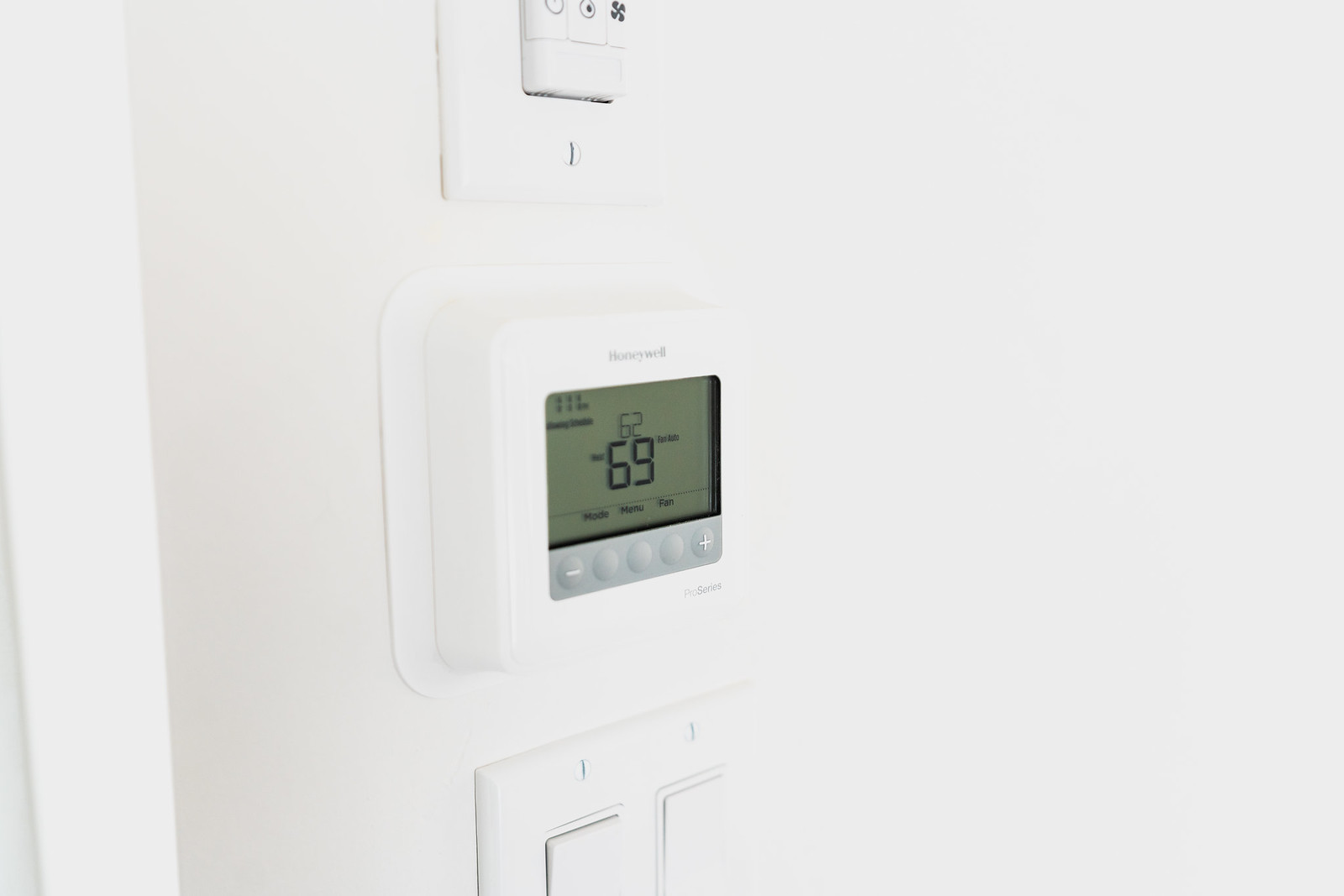A Honeywell thermostat is mounted on a wall, currently displaying a temperature of 69 degrees Fahrenheit. Below the thermostat, there is a light switch. The thermostat is part of a system that maintains the overall ambient temperature at 62 degrees Fahrenheit. The simple design and placement exhibit an efficient layout for residential temperature control.